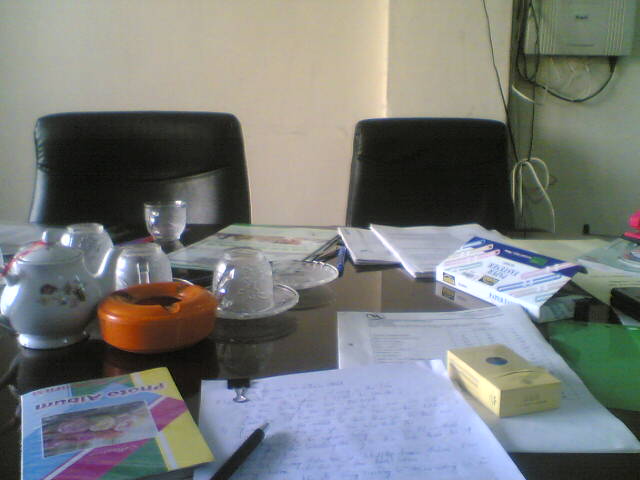The image depicts a cluttered yet organized desk with two black chairs against an off-white wall. The desk surface, which appears to be black, hosts a variety of items starting from the center and moving outward. There are several papers scattered with cursive handwriting, secured by a black office paper clip with a pen resting on top. Adjacent to these papers on the left is a book labeled "Photo Album," with an upside-down photograph partially visible on top of it.

Moving to the right, there is a light yellow, cigarette box-shaped object, possibly not actual cigarettes, perched atop what looks to be a bank statement. Further to the right, a container possibly filled with pens is present. Towards the closer end of the desk are a few coffee mugs, a teapot, and an orange ashtray, adding to the clutter.

In the background, apart from the chairs, we notice a power box affixed to the wall with black and white wires running in and out, possibly for electricity or Wi-Fi. Barely visible to the far right is a pink object, likely an office tool such as a stapler. The overall scene is a snapshot of a busy workspace, detailed with personal and office-related items.